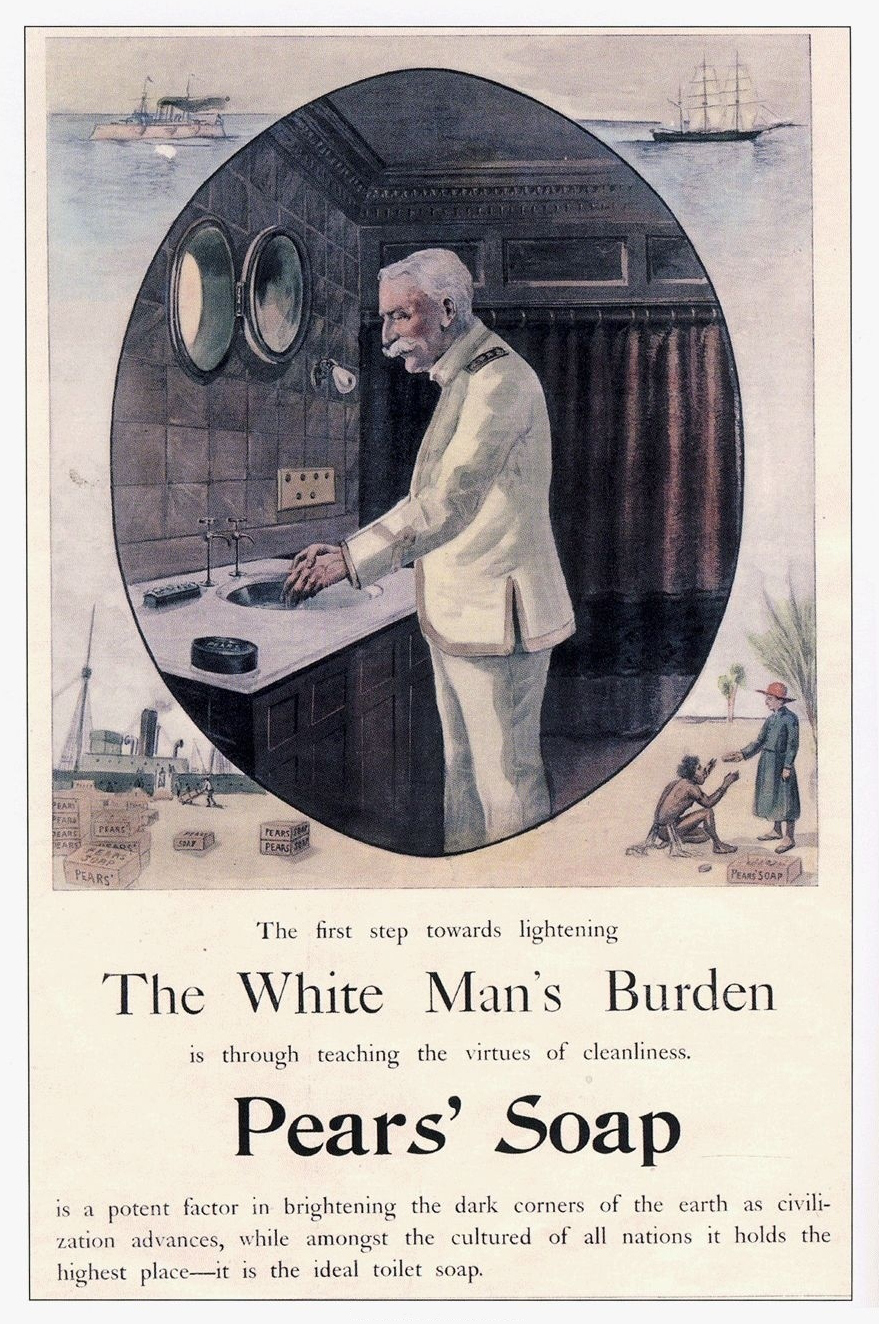The image is an old-fashioned advertisement for Pears' soap, illustrated in a vintage style. The advertisement is divided into two main sections: the top part features multiple images, and the bottom part is text.

The focal point of the upper section is an oval illustration of a sailor in a bathroom, washing his hands in front of a porthole window. He is dressed in a white sailor's uniform with insignia on his shoulder, and there is a black dish, possibly containing soap, on the counter next to him. Behind him is a red and black shower curtain. Surrounding this central image are additional graphics: at the top, there are two separate images of ships at sea. At the bottom left, a boat is docked with packages, including shipping containers being unloaded, likely containing Pears' soap. To the bottom right, there is a depiction of a woman wearing a red hat and a blue dress, handing a bar of soap to a Native man dressed in a loincloth and seated on the ground.

The text below these images reads, "The first step towards lightening the white man's burden is through teaching the virtues of cleanliness. Pears' soap is a potent factor in brightening the dark corners of the earth as civilization advances, while amongst the cultured of all nations, it holds the highest place. It is the ideal toilet soap."